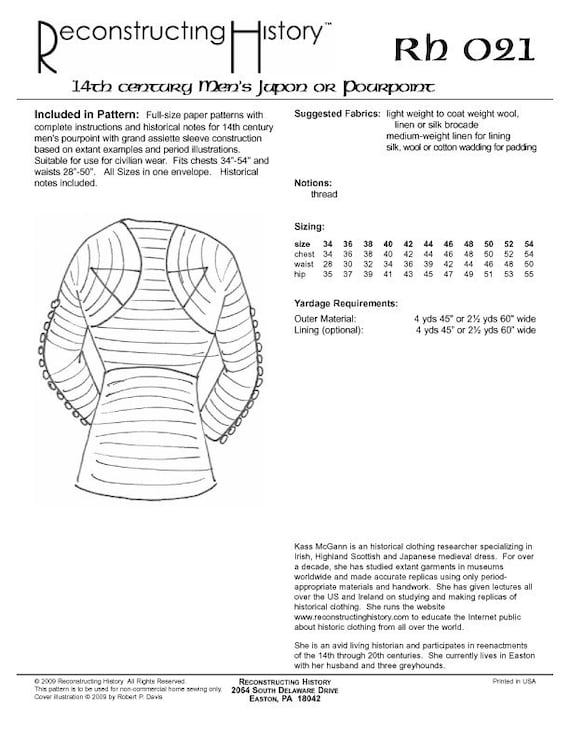The image is a meticulously detailed black and white page from a 2009 publication titled "Reconstructing History". It prominently features a comprehensive guide on making a 14th-century men's jupon or pourpoint—a type of upper body garment. The top of the page reads "Resurrecting History" and identifies the pattern as RHO21. This page includes full-size paper patterns and complete instructions, along with historical notes on the garment, which is characterized by grand asslet sleeve construction inspired by period illustrations. The pattern fits chest sizes from 34 inches to 54 inches and waist sizes from 28 inches to 50 inches, all available in a single envelope. Detailed drawings show the embroidered sleeves and ribbed material, as well as the different sizing measurements. The bottom of the page provides the contact information: Reconstructing History, 2064 South Delaware Drive, Easton, PA 18042.